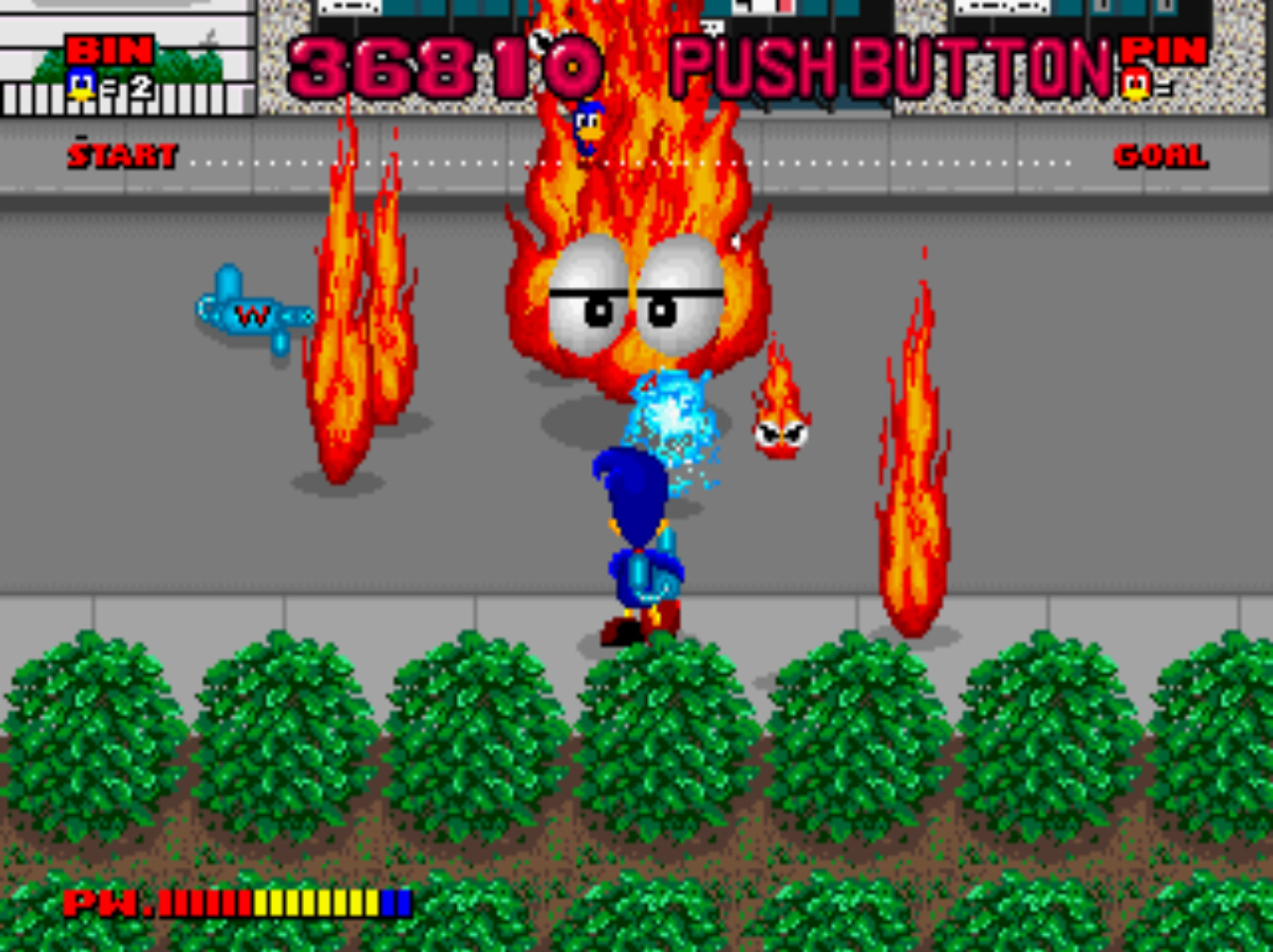In this captivating scene reminiscent of a retro pixelated video game, the spotlight is on a dynamic blue bird character clad in red shoes and equipped with a right-arm weapon connected to his backpack. Demonstrating fierce determination, he fires a blue projectile at a menacing enemy—a large flame spirit swathed in red, orange, and yellow hues, adorned with half-lidded white eyes and black pupils. Adding to the intensity, a smaller, angrier flame spirit with diagonally positioned eyelids and black pupils hovers nearby to the right. Surrounding them are three additional fires—one on the right and two on the left, devoid of any facial features.

Adjacent to one of the left-side fires lies a weapon marked with a red 'W' on its blue surface, hinting at potential power-ups. The lower portion of the image features two rows of green bushes rooted in brown dirt. The bottom-left corner displays a sequence of characters: 'P, W' followed by a red dot, leading into vertically oriented rectangles transitioning from red to yellow, and culminating in two blue rectangles.

At the top of the image, the words 'bin' and a small figure resembling a face adjacent to 'equals two' and 'start' are visible. Farther right, the number '36,810' is followed by the command 'push button,' all rendered in pink. Another 'pin' in red appears on the right with 'goal' beneath it, alongside a red spirit marked with an equal sign. Below these, the phrases 'start' and 'goal' are interspersed with white dots and centered with a blue spirit.

The epic battle unfolds on a street setting, with the protagonist positioned on the sidewalk, mirrored by a background sidewalk and building. This intricate scene captures both the nostalgic essence and the thrilling action of vintage gaming.